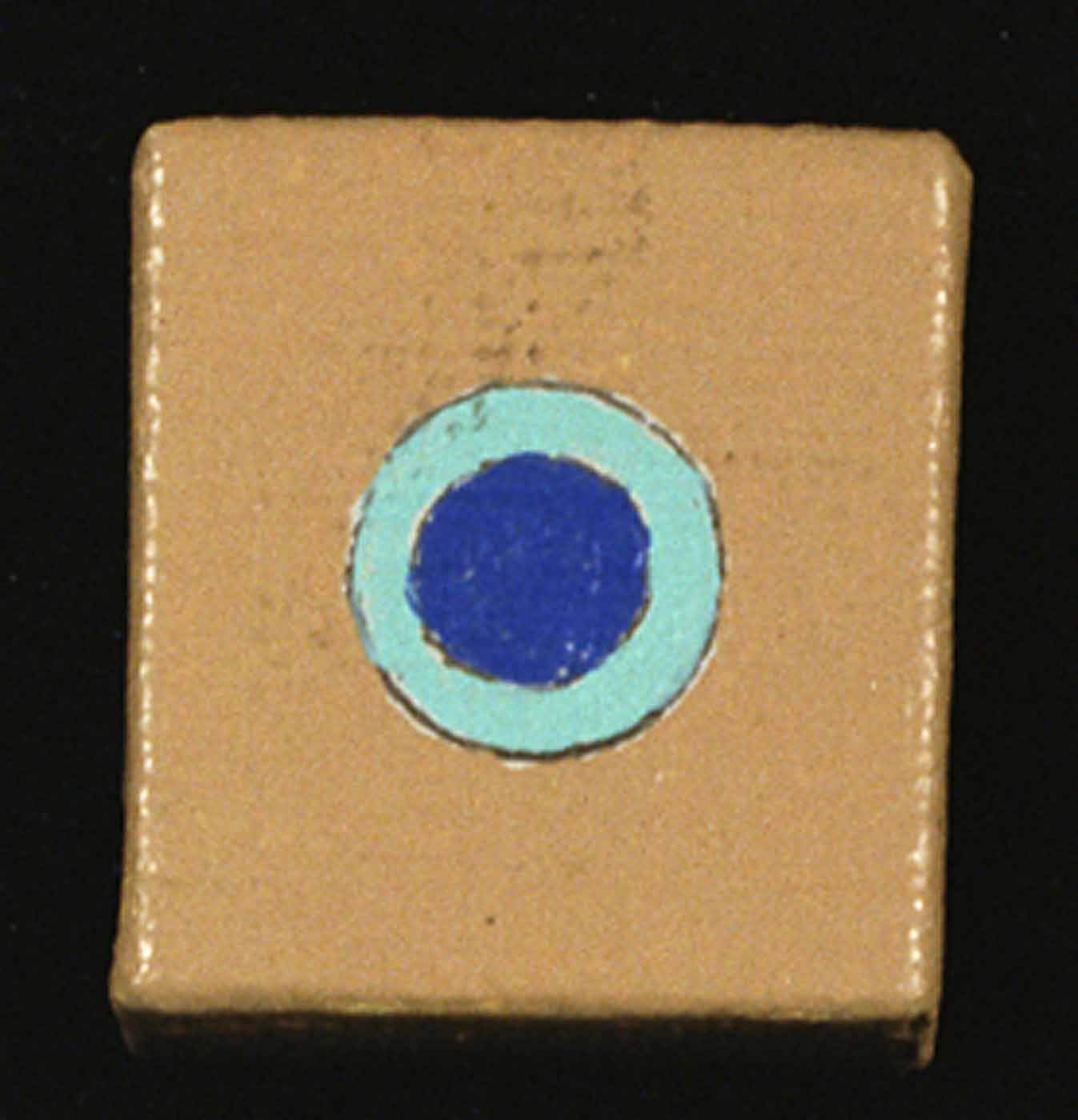This image features a centrally placed, slightly canted, square object with a shiny, almost cardboard-colored brown surface. Set against a stark black background, this brown square exhibits spots of darker pigmentation and areas of what appears to be paint wear. Lining the edges of this brown square are subtle reflections, possibly from gold paint or light glints, running vertically down either side.

Dominating the central area of the brown square is a striking circular motif. This consists of two concentric circles: the outer circle, outlined in black, is filled with a vibrant teal or turquoise blue, and the inner circle, also black-bordered, boasts a deep royal blue hue. The alignment of these colors evokes the pattern of the "evil eye" commonly seen in Greek culture, where shades of turquoise and royal blue traditionally represent protection and ward off negative energy.

The overall composition of the image, with its rich color contrasts and layered geometric shapes, presents a visually compelling and abstract aesthetic reminiscent of both cultural symbolism and modern artistic expression.